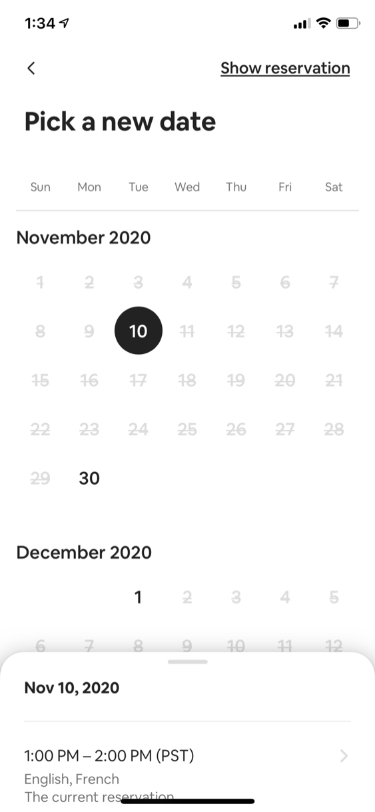A screenshot displays an online show reservation system. At first glance, it resembles a typical calendar, but a closer inspection reveals the heading "Show Reservation" at the top. Underneath, there's a bold black option labeled "Pick a New Date." The calendar layout features days of the week, from Sunday to Saturday, and the dates are highlighted in light blue. The calendar’s header reads "November 2020" in bold black. The dates, numbered from 1 to 30, are in light blue, with notable exceptions: the 10th has a bold black circle around a white number, and the 30th is in bold black text. Below the November calendar, there is a smaller section labeled "December 2020," with the number 1 in bold black. 

Below the calendars, another section appears almost like a new tab or a separate overlay, showing details for a specific reservation. It states: "November 10th, 2020, 1pm to 2pm Pacific Standard Time, English/French, Current Reservation," followed by a censored black bar concealing additional information. 

The detailed layout and highlighted dates suggest a focus on scheduling, likely indicating the significance of the listed events or reservations.